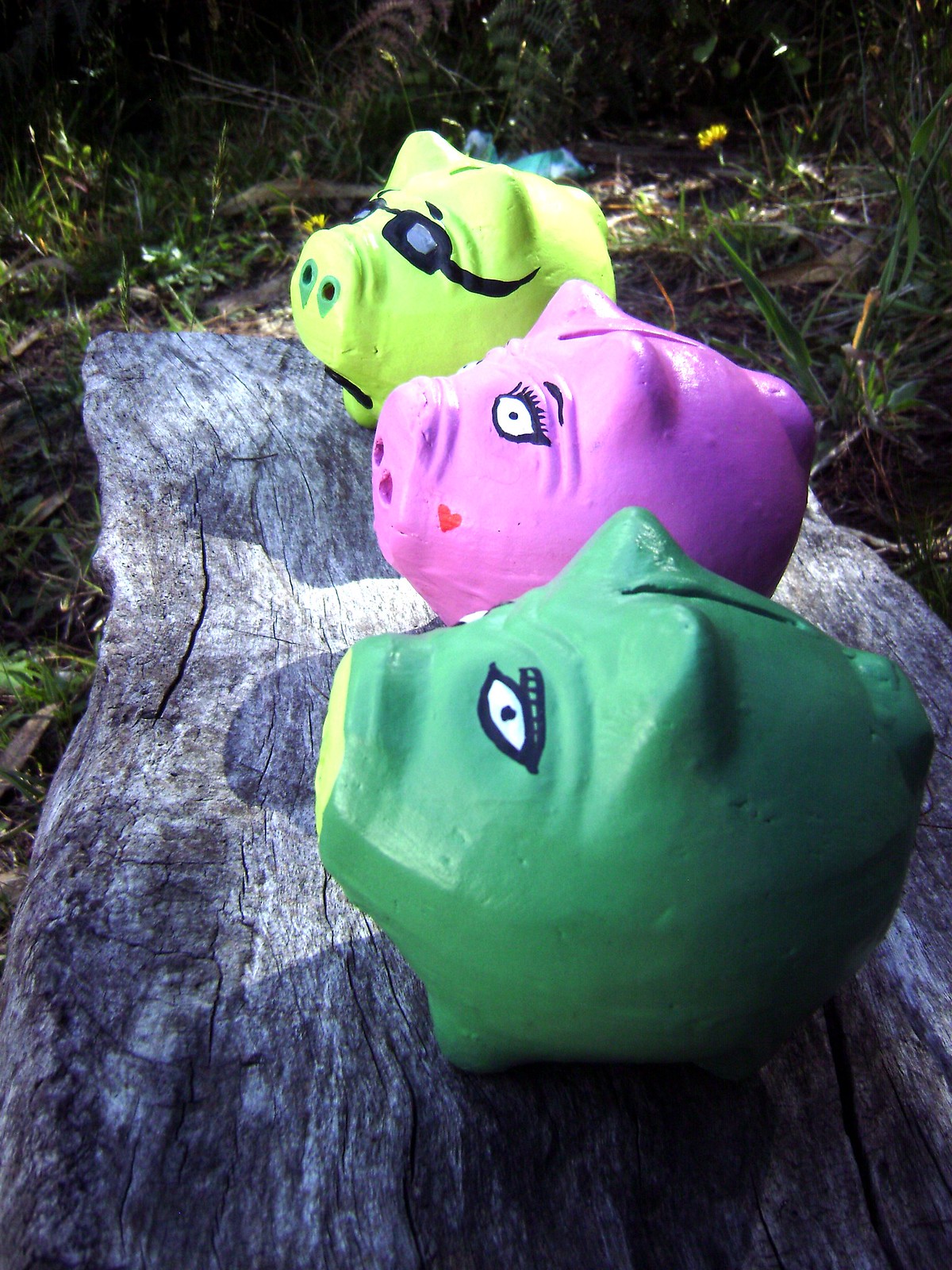The image depicts three hand-painted piggy banks arranged from back to front, perched on a grayish, flat, unfinished wooden surface outdoors. In the upper part of the image, vibrant green grass and a small yellow dandelion to the right of the rearmost piggy bank provide a natural background. The piggy bank in the back is yellow with black and gray painted sunglasses. The middle piggy bank is a striking bright pink, adorned with wide eyes, long eyelashes, and a small red heart near its snout. The frontmost piggy bank is a dark green color, featuring a light green snout and a distinctive yellow mark on the front that resembles an eyebrow. All three piggy banks are unbroken and have coin slots at the top. Despite their varied colors and designs, they are similarly sized and shaped.